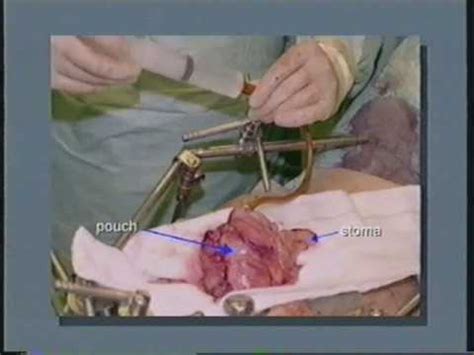The image depicts a detailed scene of a surgical procedure in a hospital setting. Central to the composition is a doctor clad in surgical gloves and gown, positioned directly in the midst of the operation. The backdrop is a dark blue color that emphasizes the sterile, controlled environment. Surrounding the surgical area are retractors and various medical instruments. The focus of the image is a diagram highlighting a pouch and a stoma, with arrows pointing to each. The stoma, a small abdominal opening used for waste removal, is prominently featured. The color palette includes shades of blue, black, green, tan, red, pink, and purple, adding to the vividness of the medical scene.